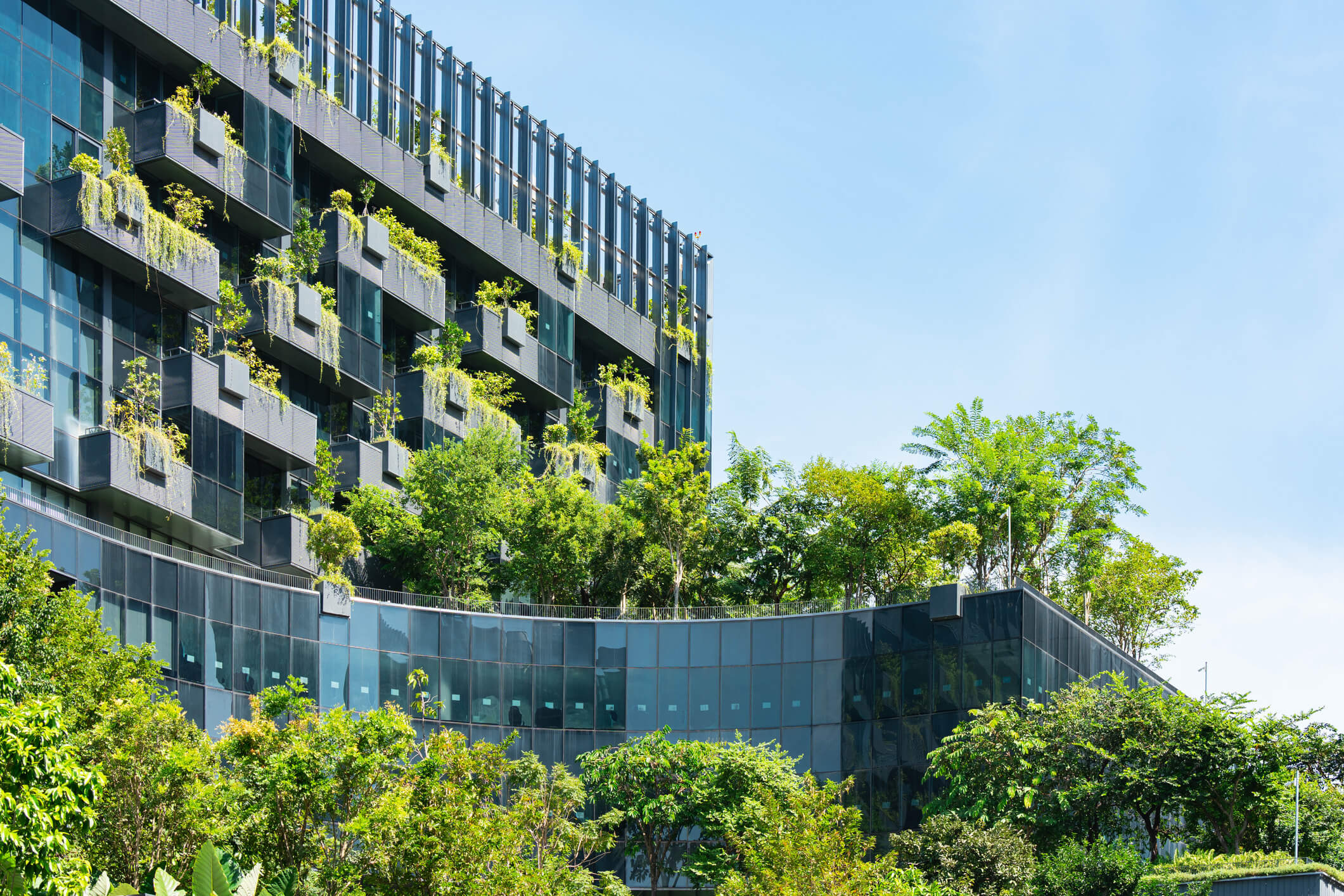The image showcases a modern, architecturally stunning building dominated by dark blue windows. The structure features two distinct sections: a taller one on the left and a shorter one on the right, the latter boasting a rooftop teeming with trees. The balconies on this building, adorned with conspicuous metal fences, are overflowing with vibrant plants, some of which cascade down in lush vines. The abundance of greenery gives the building a jungle-like appearance, suggesting it has been embraced by nature. The bottom of the image reveals a curved glass wall, slightly bluish, behind which four floors of terraces are visible, each with various green and yellow plants spilling over. Above the main structure, a beam extends diagonally, and a fence lines the top of the taller section, adding to the intricate design. The scene is set against a glowing, sunny sky with wispy white clouds, highlighting the modern yet nature-infused essence of the building.